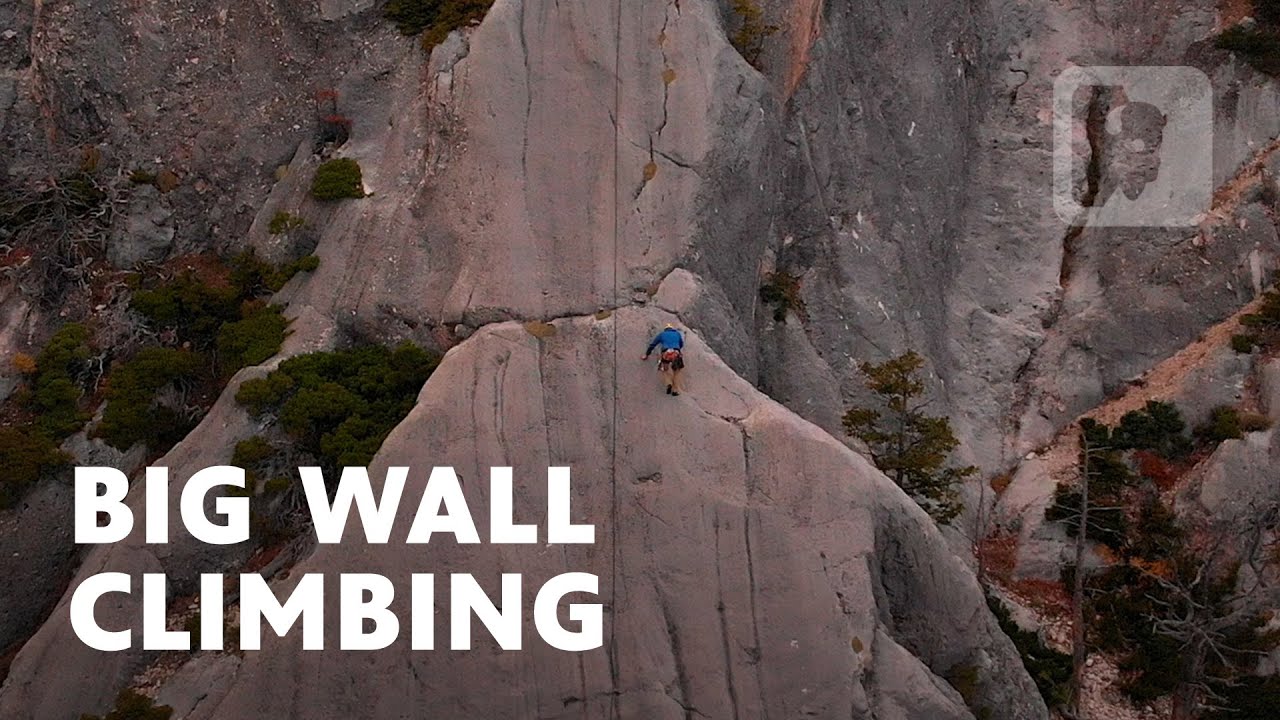The photograph depicts a distant rock climber, whose gender is indeterminate, scaling a steep, jagged rock wall. The climber, about halfway up the formidable rocky surface, is adorned in a long-sleeved blue shirt, khaki pants, and a white hardhat helmet. They appear to be equipped with a backpack and climbing gear, although specific ropes or harnesses are indiscernible. The landscape features a mix of green shrubs and trees, interspersed with some dead pine trees at the base. The rugged rock face exhibits hues of pink, gray, and brown, with a smooth yet cracked surface where the climber ascends. Bold white text in large capital letters at the bottom left corner reads "BIG WALL CLIMBING." A translucent gray square with a cut-out image of a buffalo head is present in the top right corner, suggesting a logo, possibly affiliated with the big wall climbing enterprise. The overall atmosphere of the photo exudes the challenge and exhilaration of outdoor rock climbing.